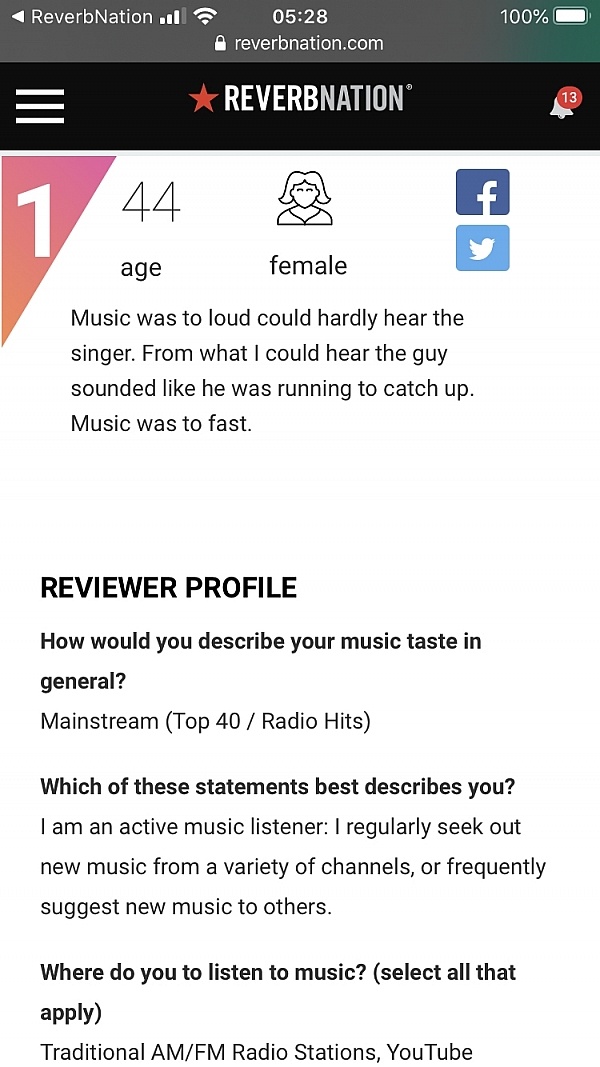The image captures a cell phone screen displaying a website called Reverbnation. At the very top, "Reverbnation" is prominently written in white. Surrounding this are various icons typical of a smartphone interface: a signal icon for phone reception, a white arrow pointing to the left, a Wi-Fi symbol, the time "05:28", and a fully charged battery icon showing 100%. Directly beneath, there's a small lock symbol followed by the website URL "reverbnation.com", all enclosed within a small, shaded area. 

Below this, the screen transitions into a black shaded area. On the left, three horizontal white lines are visible, indicative of a menu icon. Centered in this area, there is a red star icon adjacent to the word "Reverbnation", both in white. To the right, a notification bell icon shows the number 13 in white, enclosed in a red circle. 

Further down, the screen presents a user profile section. On the left, a small black triangle pointing downward sits beside the number 1 and the number 44, followed by the text "age". A black and white icon of a woman indicating "female" is directly below this, with adjacent icons for Facebook (a white "F" on a blue square) and Twitter (a white bird on a blue square).

Expanding on the profile's content, it reads: "Music was so loud could hardly hear singer. From what I could hear the guy sounded like he was running to catch up. Music was too fast." This reflects a user's review on the platform. The section continues with questions and answers about the user's music preferences. The user describes their music taste as "mainstream top 40 radio hits" and identifies as "an active music listener" who regularly seeks out new music and frequently suggests it to others. For listening habits, the user selects "traditional AM/FM radio stations" and "YouTube."

The entire screen is set against a plain white background, ensuring all text and icons are easily legible.